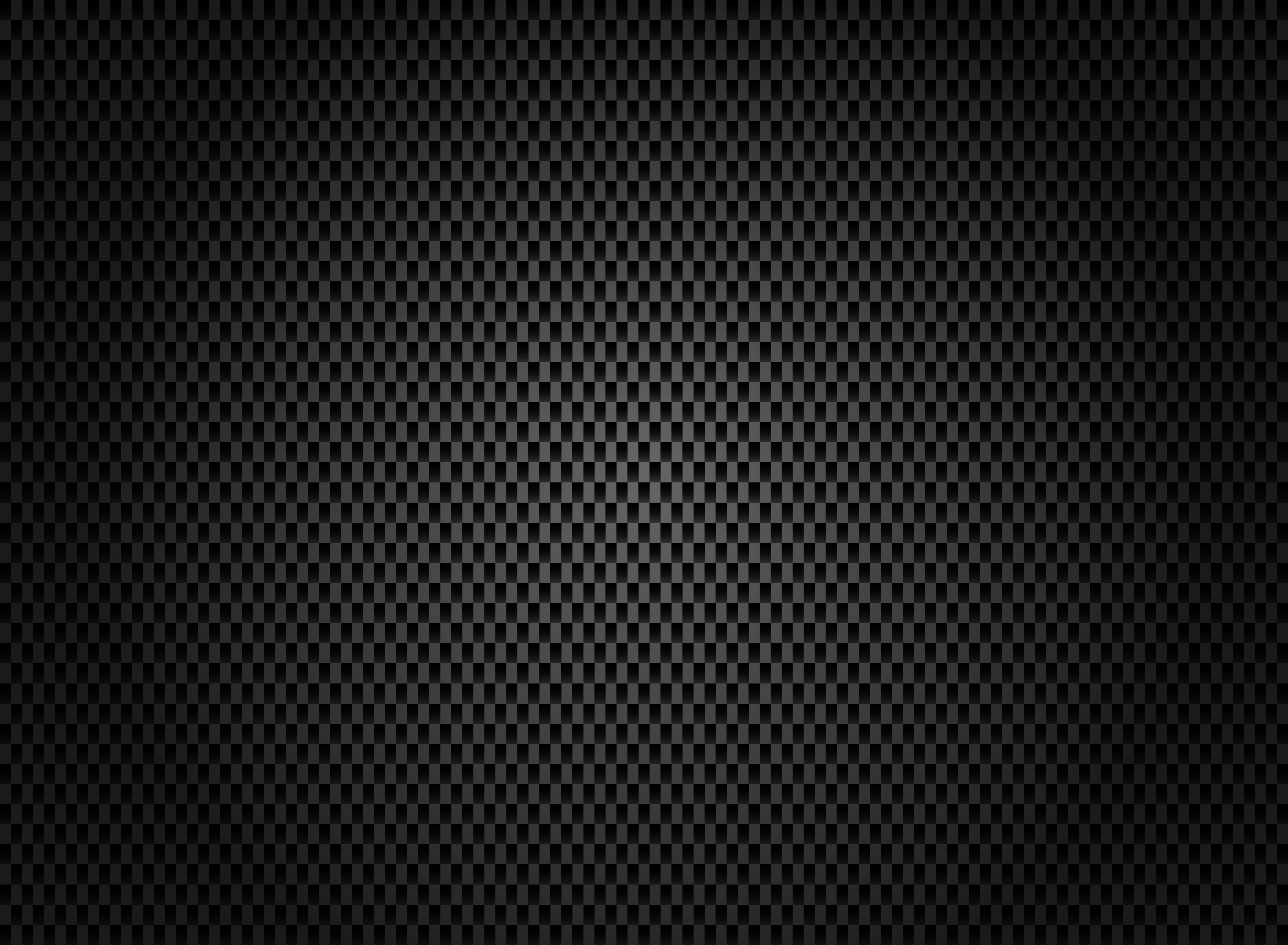The image is a two-tone, computer-generated geometric illustration in a rectangular, landscape orientation. Composed of hundreds of tiny black and gray rectangles, densely arranged in a grid pattern, the individual rectangles measure a few millimeters in height and width, creating an intricate optical illusion. Although the pattern alternates between black and varying shades of gray, the intensity of the gray shades shifts towards the center. This gradient effect causes the central area to appear as though it is illuminated by a bright, glowing orb, creating a visual contrast where the middle is lighter and the edges gradually become darker. The entire image, resembling a tightly compacted chessboard or a pattern composed of countless small elements, gives the illusion of light shining from the center, creating a dynamic and captivating visual impact.